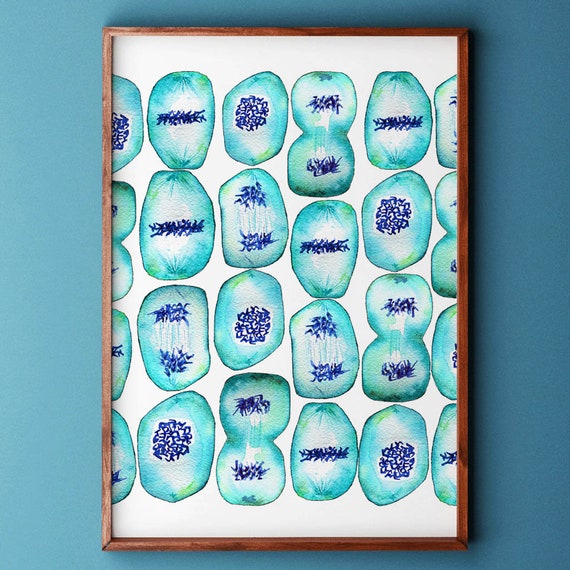The image depicts a framed artwork hanging on a light blue wall that deepens in color from left to right. The frame itself is a thin, brown wooden rectangle, slightly taller than it is wide. Inside the frame, the artwork features a white background adorned with numerous green, oval-shaped blobs. These blobs, which have unique and irregular shapes, resemble the random splatters of a liquid. Each blob contains intricate blue scribbles, many of which form what appear to be chromosomes, indicating a biological theme, possibly representing cells undergoing mitosis or meiosis. The artist has carefully positioned at least 20 or so of these cell-like figures side by side, creating an intriguing visual pattern that emphasizes the dynamic nature of cellular structures.